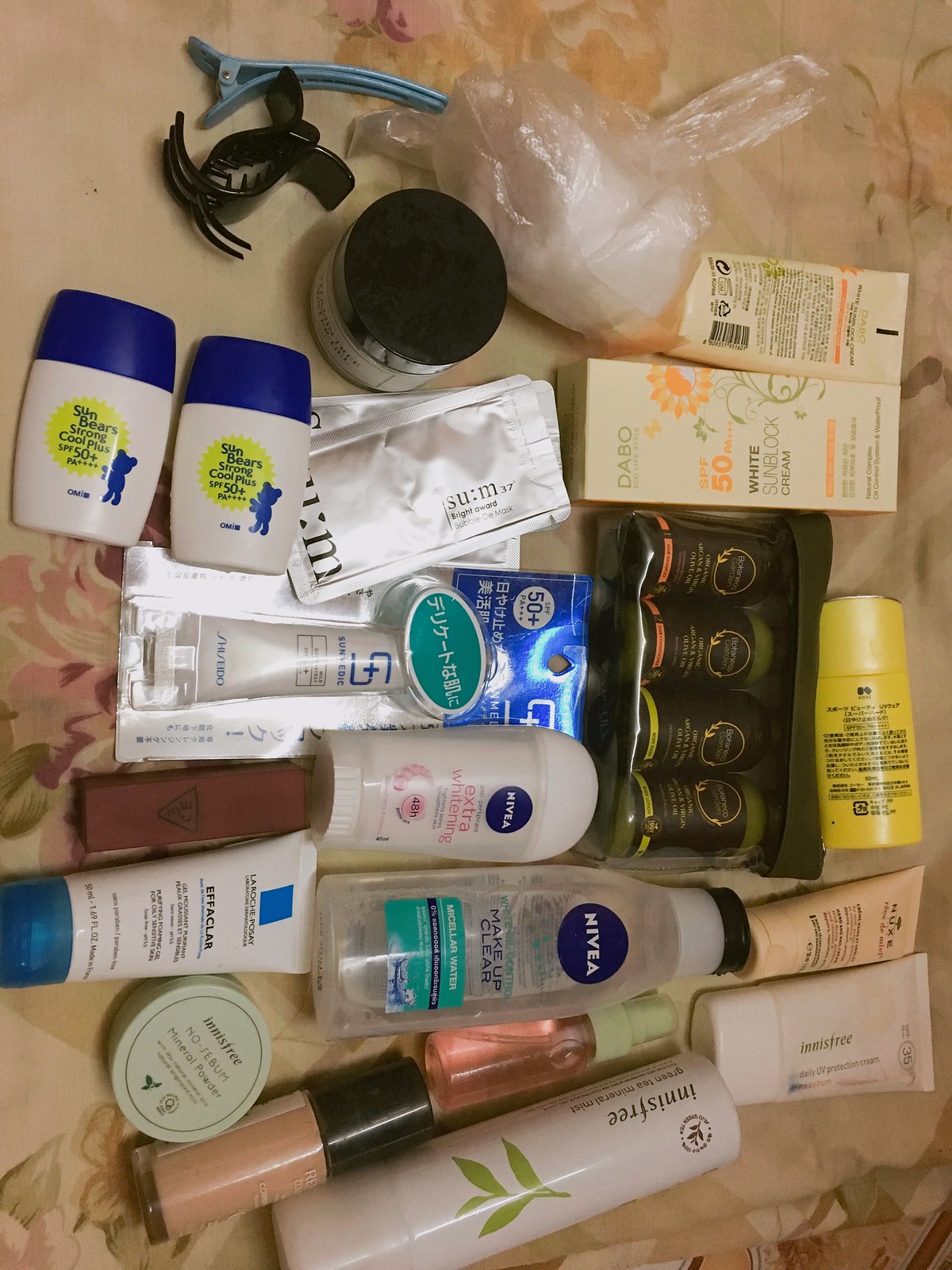The photograph, rotated to its side, showcases an array of cosmetic and personal hygiene products meticulously arranged on a beige and brown floral-patterned comforter. Positioned at the upper center of the image, a blue curved hair clip and a brown claw hair clip draw the eye. Adjacent to these clips on the right is a plastic bag containing a white item, with its handles tied and angled towards the top right corner of the photo. 

In the upper left region, two slightly oval containers of a product named "Sun Bear" are visible, characterized by a flattened top and bottom and a distinctive design featuring a blue silhouette of a small bear and a yellow sun at the center. Nearby, a rectangular transparent container of Nivea Makeup Clear stands out, with its cylindrical top leading into the rectangular base and the iconic round Nivea emblem showcasing the brand name in white letters. Finally, completing the collection is a cylindrical container from Innisfree, adorned with a green leaf design, located towards the left side of the arrangement.